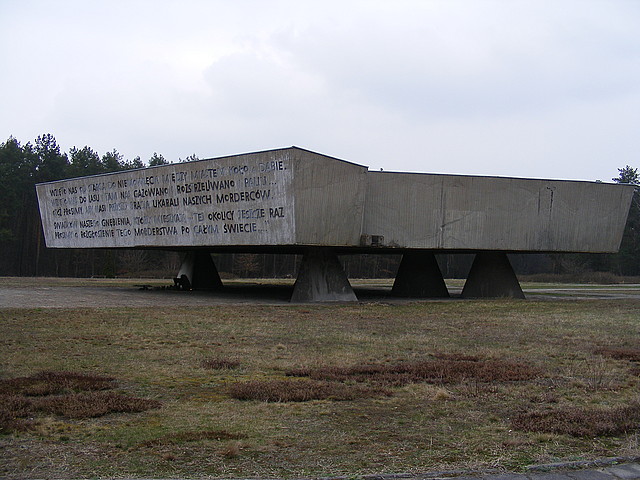This is a photo of a large, austere concrete sculpture arranged in a rectangular, L-shaped formation. The sculpture is primarily composed of two attached trapezoidal segments, extending toward the left and right sides of the image, respectively. It rests on four sizable triangle-shaped bases, lending an asymmetrical and industrial aesthetic to the structure. The front face of the sculpture is etched with five lines of text in a non-English language, possibly Russian or Polish, utilizing a blocky, all-caps font that spans the entire surface. The photo was taken on an overcast day, with clouds casting a gray-blue hue over the scene. In the background, there are tall evergreen trees, while patches of dead grass with sparse green tufts lay in the foreground.